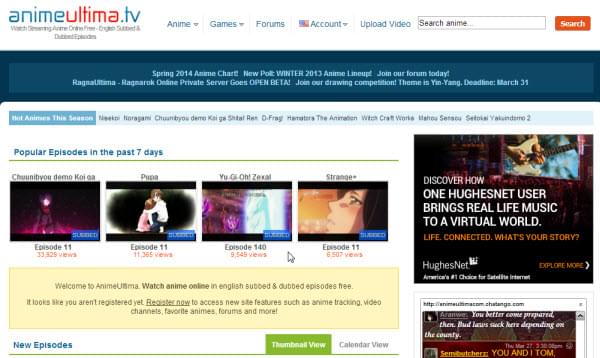A landscape screenshot from the website AnimeUltima.tv is meticulously captured in this detailed description. In the upper left-hand corner, the website’s name "animeultima.tv" is prominently displayed. The upper center section features category headers such as "Anime" with a dropdown menu, "Games" with a dropdown menu, "Forums," and "Account," which is accompanied by an American flag and a dropdown menu. Adjacent to these headers is a button labeled "Upload Video," followed by a search bar that prompts users to "Search Anime." In the upper right-hand corner, a red "Search" button is clearly visible.

The main content area is divided into sections, beginning with a dark blue banner displaying options like "Spring 2014 Anime Chart," "New Poll," "Winter 2013 Anime Lineup," and "Join Our Forum Today." Due to the resolution, some of the text in this area is unreadable. 

Below this banner is another section with a white background, showcasing "Popular Episodes in the Past Seven Days." This section includes anime thumbnails with titles overlaying them, though only the fourth thumbnail's title is legible, reading "Strange." Beneath each thumbnail are episode indicators: "Episode 11," "Episode 11," "Episode 140," and "Episode 11," respectively.

This elaborate screenshot encapsulates various facets of the AnimeUltima.tv website, offering a comprehensive view of its layout and content.